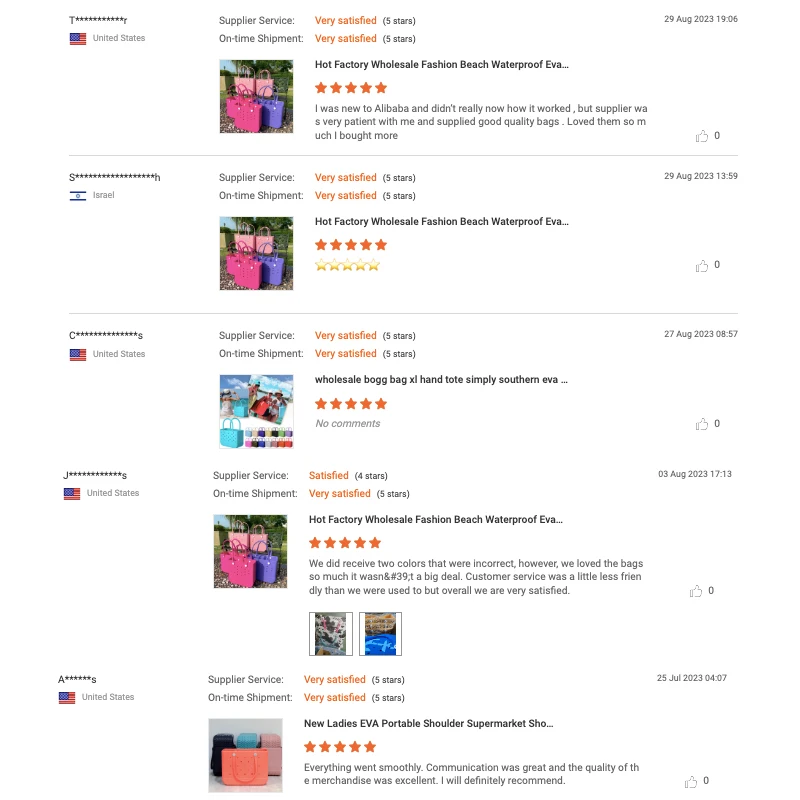This image appears to be a tablet screenshot showcasing a feedback system on a shopping platform. The screen displays a list of user reviews for various products, primarily bags and accessories. Each review is formatted within a horizontal section, separated by thin lines.

### Detailed Description:
- **Background and Layout**: The overall background is white, creating a clean, uncluttered view. The layout uses a series of horizontal sections to organize information neatly.
- **Usernames and Locations**: The leftmost column lists usernames that are partially obscured for privacy, displaying only the first letter followed by a series of asterisks (e.g., J*****). Accompanying each username is a small icon representing the reviewer's country: predominantly the United States, with one from Israel.
- **Feedback Details**: Alongside the usernames, feedback sections comprise several components: supplier service satisfaction and on-time shipment ratings, both of which are represented with star ratings. Each feedback entry includes a small thumbnail image, likely depicting the reviewed item.
- **Product Information**: The products being reviewed include various bags and accessories. Sample product names include “Hot Factory Wholesale Fashion Beach Waterproof Cut-off Something" and "Wholesale Bug Bag Hand Tote Simply Southern." The descriptions suggest these items are fashion-related, emphasizing portability and style.
- **Ratings and Reviews**: Each feedback segment permits users to rate various aspects of the purchase, primarily focusing on supplier service satisfaction and the timeliness of the shipment. Stars filled in or left empty indicate the level of satisfaction.

This screenshot encapsulates a user-friendly interface for collecting and displaying feedback on a shopping platform, allowing for an organized look at customer satisfaction regarding product and service quality.